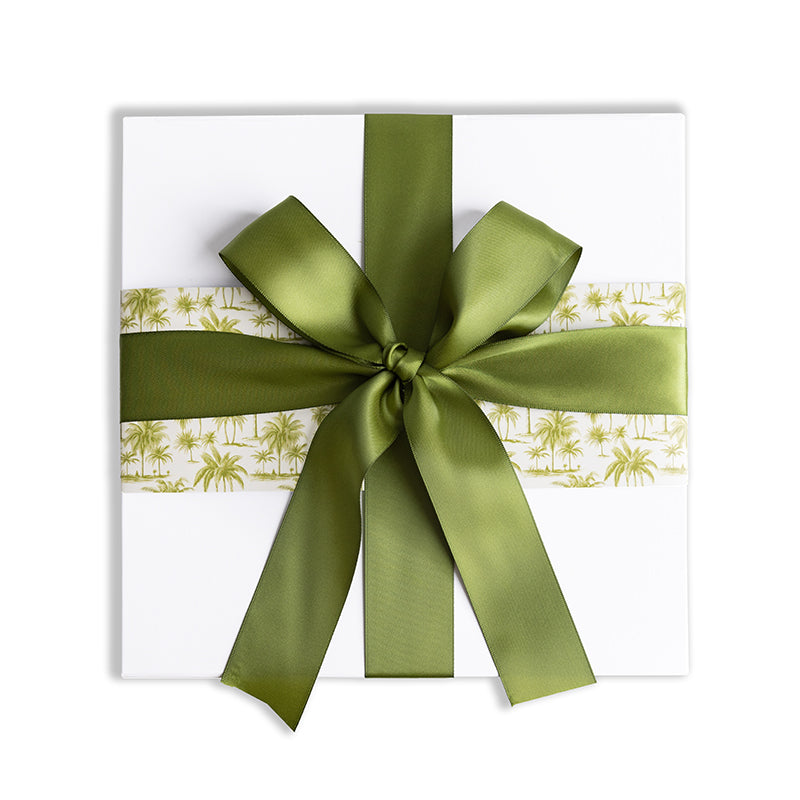The photograph showcases a pristine white, square gift box adorned with an elaborate green ribbon. The silky ribbon is tied in a lush bow at the top and extends vertically and horizontally around the box. Across the center of the box, a cream-colored band features a pattern of green palm trees of varying sizes, some accompanied by patches of grass, adding a tropical touch. The box sits against a seamless white background, casting a faint shadow to its left and top. The design is clean and uncluttered, with no labels or additional markings, emphasizing the elegant simplicity of the wrapping.